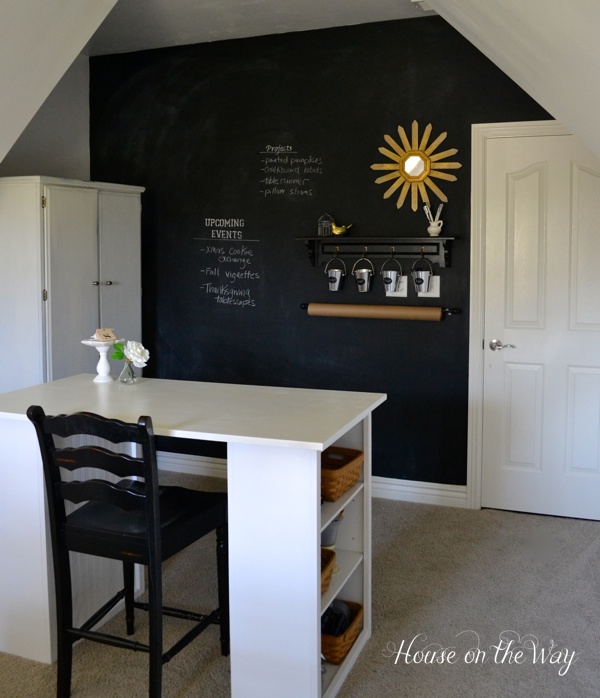This image captures a meticulously organized multi-purpose room within a home, possibly doubling as a kitchen, dining room, or craft area. Dominating the scene is a white central table with multiple shelves, each filled with baskets for craft supplies. A high black chair sits invitingly at the table, which is adorned with a white rose sculpture and a white centerpiece.

The back wall of the room is painted in chalkboard black, allowing for handwritten notes and schedules. The writing on the wall is neatly divided into sections labeled "Upcoming Events" and "Projects," listing various activities like "Christmas Cookie Exchange," "Fall Vignettes," and "Thanksgiving Tabletops." In addition, the wall showcases whimsical drawings, including a sun, and practical elements like a hanging shelf with silver buckets, each possibly assigned a name.

To the right of this chalkboard wall is a pristine white door with a silver handle. Adjacent to the door, a mirror shaped like a daisy or sun adds a decorative touch, under which two shelves hold various items including silver watering cans hanging by hooks and a roll of wrapping paper. Further to the side, a white cabinet with two doors stands against the wall. A subtle watermark reading "House on the Way" is also visible in the image.